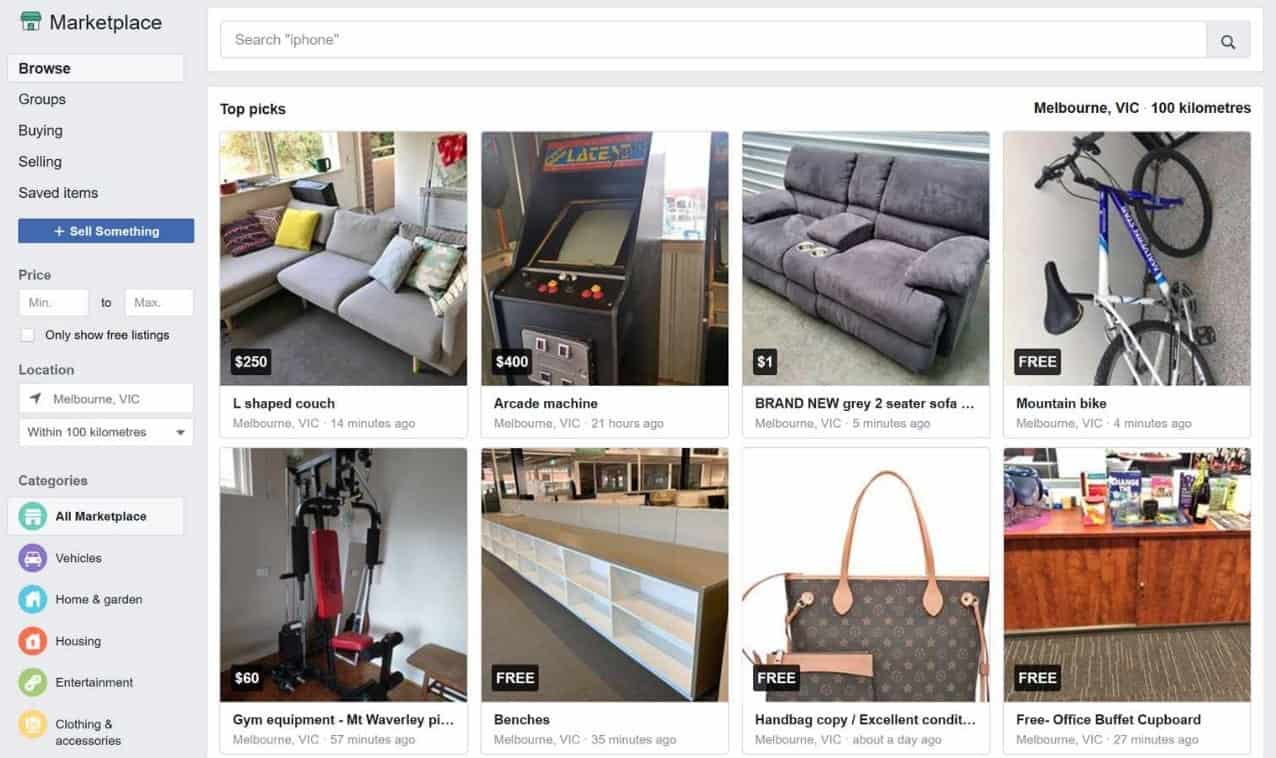The image depicts a webpage for an online marketplace with a focus on a detailed user interface. At the top left of the page, there's a shadow-gray box labeled "Flag as Inappropriate." Below this box, there is an inventory list with the heading "Marketplace," accompanied by a green icon resembling a store with a green roof.

The inventory list includes several categories: "Browse," "Groups," "Buying," "Selling," "Saved Items," and a clickable "Sell Something" button. Users can filter items based on price ranges, including "Price from Minimum to Maximum," and can opt to view "Only Show Free Listings." Additional filters include geographical location ("Within 100 kilometers"), and various item categories such as "All Marketplace," "Vehicles," "Home," "Garden," "Housing," "Entertainment," and "Clothing and Accessories."

To the right, there is a search bar with an adjacent hourglass icon. The central part of the page features eight photos under the heading "Top Picks." These images showcase a variety of items available for sale in the Melbourne area within a 100-kilometer radius.

The items include:
1. A sofa priced at $250
2. A gaming console for $400
3. A brand new gray two-seater sofa for $1
4. A blue and white mountain bike available for free
5. Exercise equipment listed at $60
6. A bench available for free
7. A high-quality handbag copy for free
8. A free office buffet cupboard

Each item is presented with a clear image, and the price or availability status is prominently displayed.